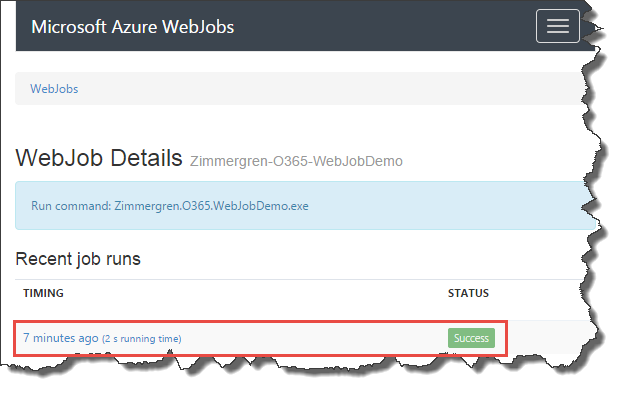In this detailed image, we observe the interface of Microsoft Azure, specifically focusing on WebJobs. At the top, various tabs are displayed, including "WebJobs" and "WebJobDetails." The highlighted WebJob is named "Xamarin-0365-WebJobDemo," with the command "Xamarin.0365.WebJobDemo.exe" executed.

Below this, a section labeled "Recent Job Runs" provides information on the job's recent execution timings: it was initiated seven minutes ago and had a running time of two seconds. The job's status is marked as "success," and this status is prominently highlighted in red. The overall color scheme of the interface features shades of gray, white, and blue, creating a clean and professional aesthetic suitable for a development environment.